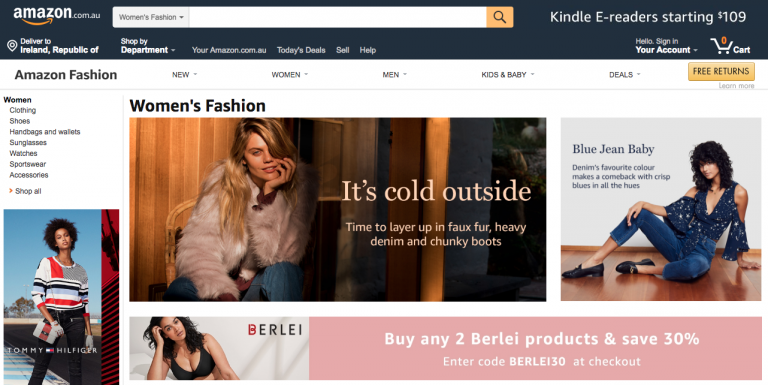This image is a screenshot from the Amazon Fashion section on Amazon.com. At the top, it features the familiar dark gray header with the Amazon logo in white, alongside the signature gold Amazon smile in the upper left corner. Below the header is a white navigational menu with categories including "Amazon Fashion," "New," "Women," "Men," "Kids and Baby," and "Deals."

The main section of the image showcases two large promotional photos. On the left, under the headline "It's cold outside. Time to layer up," the image highlights styles like faux fur, heavy denim, and chunky boots. The model, a white woman with long blonde hair, is shown wearing a white faux fur jacket and denim jeans.

On the right, another headline reads "Blue Jean Baby." This section features a model sitting on the floor, a white woman with curly dark brown hair. She is dressed in denim skinny jeans and a denim halter top with polka dots.

At the bottom of the image, there is a pink rectangle with white text announcing a special offer: "Buy any two Belei products and save 30%." To the left of this text is a photo of another model, a white woman with dark hair, wearing a black bra.